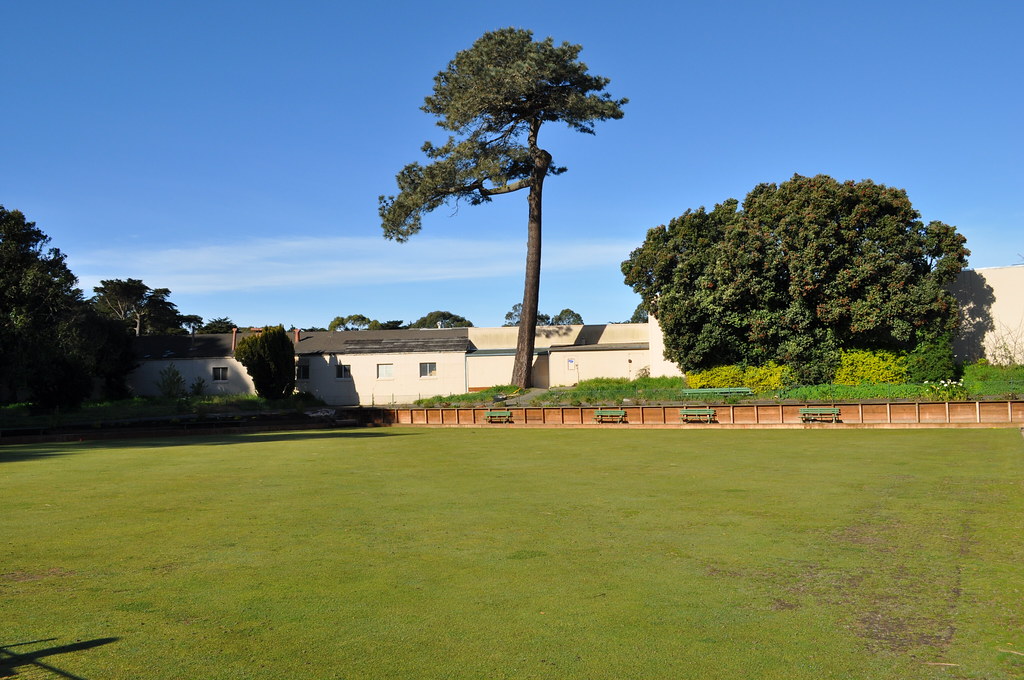The photo depicts a sunny, daytime scene of an unmarked grassy field, possibly used for soccer or football. The sky occupies the upper half of the image and is a clear blue with a streak of white mist near the horizon. The field is bordered by a row of four green benches positioned along a wooden berm, situated near the rear of the field. Behind the benches, there is a tall tree and a shorter, wider tree or bush. To the left, the landscape features more tree growth, casting shadows across the field. On the right side of the image, partially obscured by trees, is a white building with a shingle roof, extending towards the center. This structure, which could be a home or part of a complex, highlights the park-like atmosphere of the scene. The grass is cut low, and the overall setting feels serene and open, with the sunlight reflecting warmly off the leaves and the field.